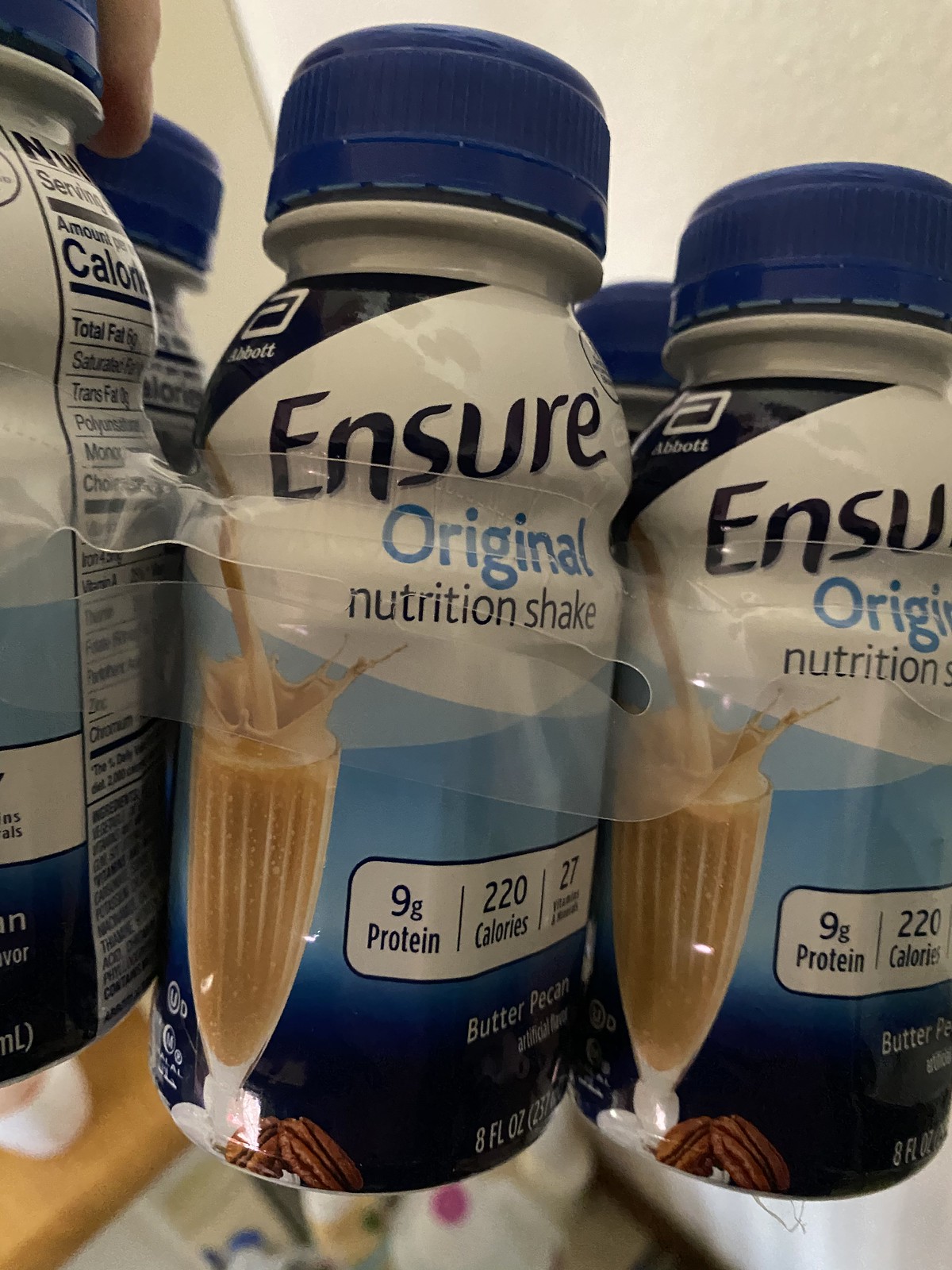A close-up photograph showcases a six-pack of Ensure nutritional shakes, although only five bottles are visible. The bottles are neatly arranged in a clear plastic holder, which is being held by a person in the upper left-hand side of the image. Each bottle features distinctive packaging elements, including a blue cap and the brand name "Ensure" prominently displayed in black lettering. Beneath the brand name, "Original" is written in blue lettering, followed by the description "Nutritional Shake" in black font.

An enticing image of a tan-brown shake being poured into a glass is depicted on the left side of each bottle; the shake overflows, creating a dynamic splash effect. The bottle also highlights key nutritional information below this image, stating that each shake contains 9 grams of protein, 220 calories, and 27 essential vitamins and minerals. The flavor is clearly labeled as "Butter Pecan" at the bottom of the bottles.

The photograph's extreme close-up perspective focuses on the intricate details of the packaging, color, and text, offering an intimate look at the product.